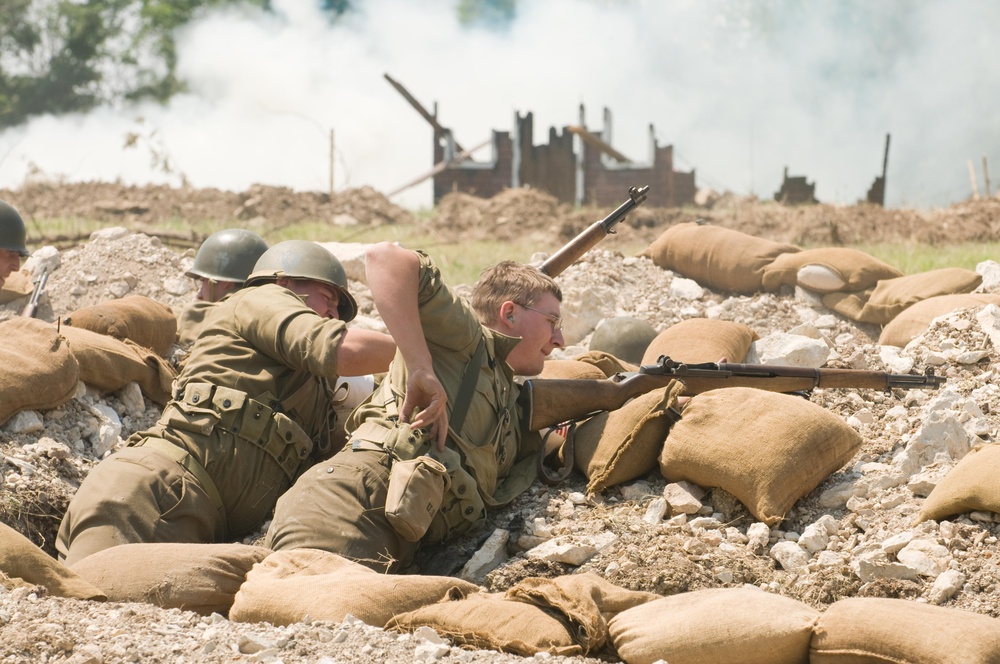This detailed photo captures a scene of military men either practicing or engaged in combat, set in a wartime environment during daylight. The central focus is on three soldiers hunkered down in a freshly dug foxhole, surrounded by dirt, white rocks, and burlap sandbags forming a defensive barrier. The soldiers are all dressed in matching green uniforms consisting of green shirts, pants, and waist bags, and two of them wear green metal helmets. Each man is armed with a rifle featuring wooden and black metal components. 

The man closest to the camera, positioned centrally, is a Caucasian soldier wearing glasses and no helmet. He is reaching into his waist bag for ammunition, and his rifle is propped up on the sandbags. The upper portion of the image is obscured by smoke, evidence of the ongoing battle. Behind the soldiers, you can see the debris of a destroyed building, and in the upper left corner, faint outlines of trees. The overall atmosphere is tense and chaotic, indicating an active wartime scenario.